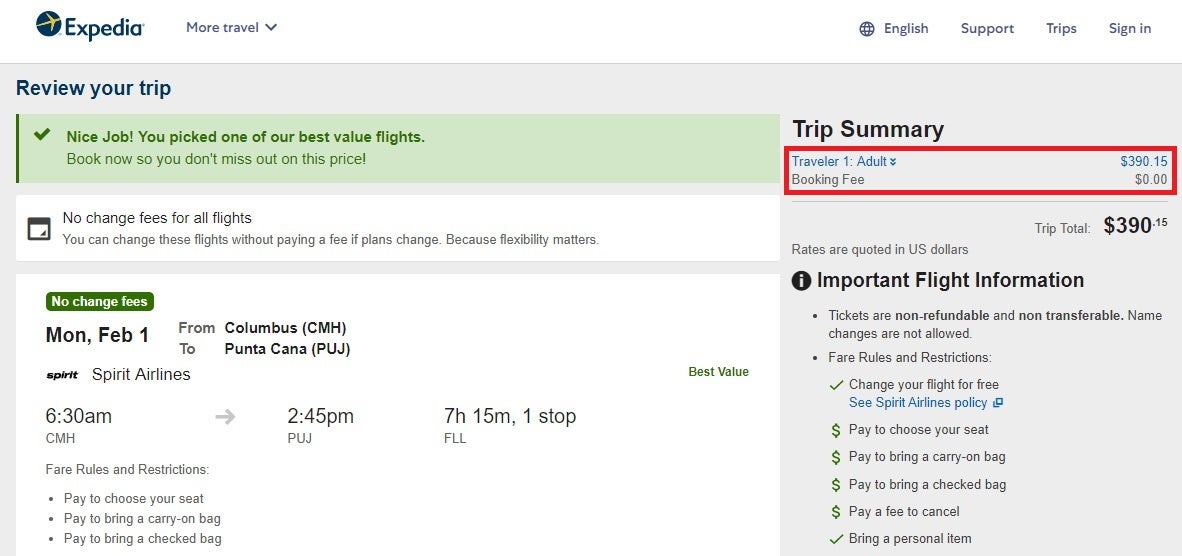This image is a cropped screenshot of the Expedia website on the "Review Your Trip" page. At the top left, the distinctive Expedia logo is prominently displayed. To its right, the phrase "More Travel" appears in small blue letters, indicating a drop-down menu that can be expanded using the adjacent arrow. 

Directly below, the page title "Review Your Trip" is highlighted in bold blue letters. Beneath this, a large green banner with a check mark on the left side enthusiastically declares, "Nice Job! You picked one of our best value flights. Book now so you don't miss out on this price." 

Following the green banner, a white one emphasizes the benefit of "No Change Fees for all flights," explaining that travelers can modify their flights without incurring additional charges if their plans change, underscoring the importance of flexibility.

Towards the bottom of the image, a large white box features a green bubble at the top, reiterating "No Change Fees." Below this, there are sections for Departure and Arrival Destinations, Spirit Airlines, and Times, which provide specific details about the flight. 

On the right side of the image, the "Trip Summary" section is displayed in bold black letters. Underneath, it lists "Traveler" and "Booking Fee," with a red box highlighting that there is a $0 booking fee and the price for travel for one adult.